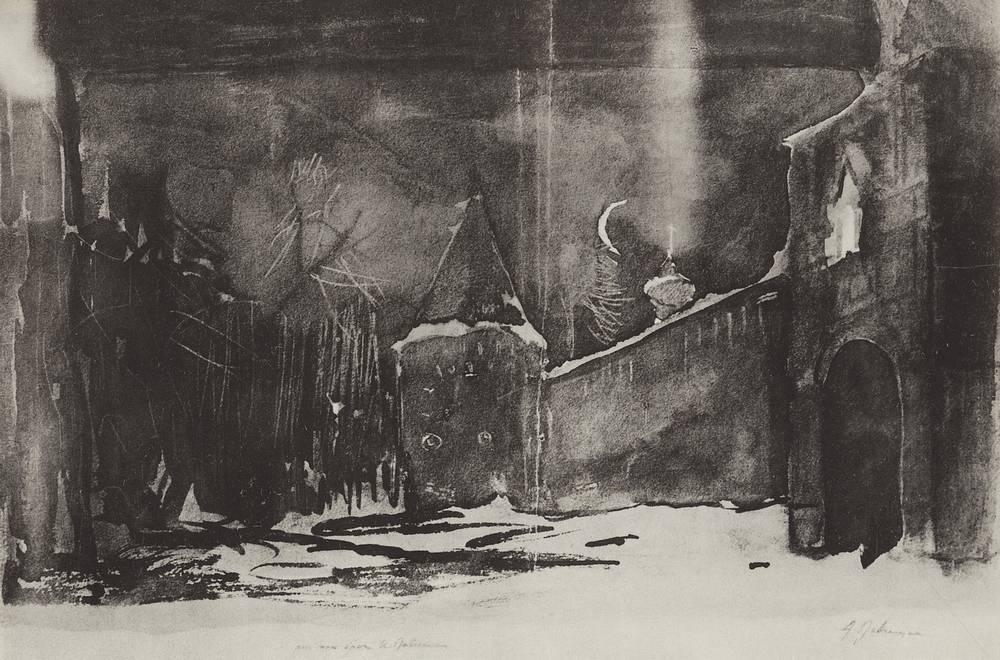This grayscale drawing renders a moody and dark nighttime scene of an ancient, possibly castle, cityscape veiled under a cold winter night with snow-covered ground. Dominating the right side of the composition is a high city wall, highlighted by a rounded gate entrance and a tall rectangular tower with an arched doorway. This tower features a triangular window near its top, adding to the medieval ambiance. The wall extends into the middle left of the drawing, shrouded in dark, shadowy tones under the night sky, from which a crescent moon glows above. In the central foreground, a mysterious pointed structure adorned with white markings stands out, possibly hinting at an important building. Sparse, leafless trees dot the snowy landscape, reinforcing the cold, barren winter setting. The entire scene is depicted without any text, emphasizing the ancient and abstract quality of this evocative, black-and-white artwork.